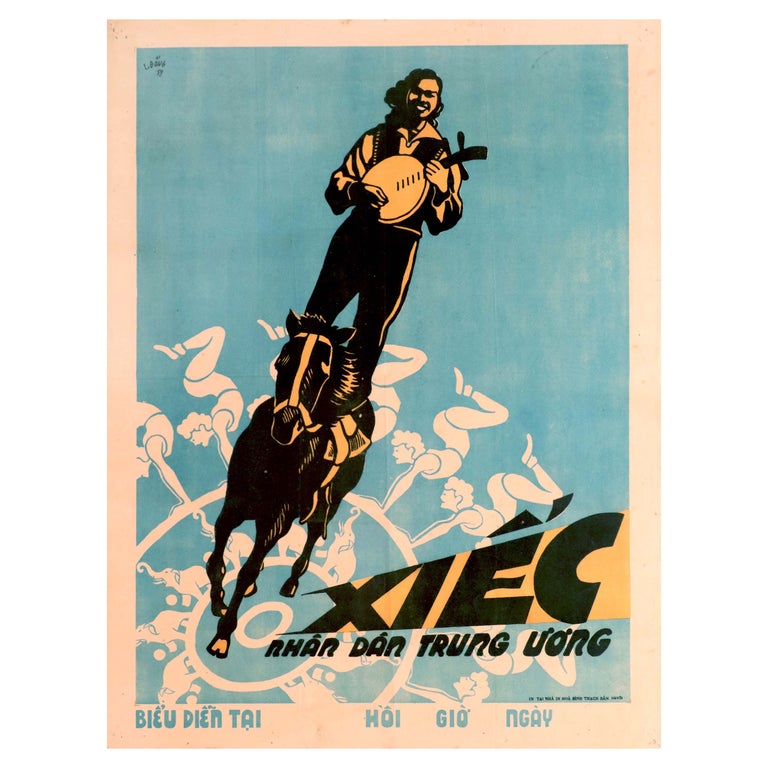The image appears to be a vintage poster, possibly for a circus or theatrical performance, featuring vivid pastel colors with a blue and white background. At the center of the poster is a striking black horse adorned with a yellow bridle and harness. Standing triumphantly on the horse's back is a man dressed in black pants, a black vest, and a long-sleeved collared shirt. The man, with long wavy hair and conspicuously yellowish skin and face, is joyfully playing a small, round instrument resembling a mandolin or a banjo.

Around the base of the horse is an intricate circular scene reminiscent of a carousel. The outer ring is comprised of women gymnasts performing handstands with bent legs, forming a visual wheel. Central to this carousel-like image are a group of elephants with their trunks raised high, enhancing the spectacular and whimsical nature of the composition.

The poster includes notations in a foreign language. Adjacent to the horse, text in black and yellow reads "XIEC. Ran, Don, Trung, Wong." Beneath this, a blue text string displays "BIEU, DIEN, TAI, HOI, GIO, NGRY." This carefully crafted and visually rich poster aims to captivate and intrigue the audience with its eclectic and detailed scene.